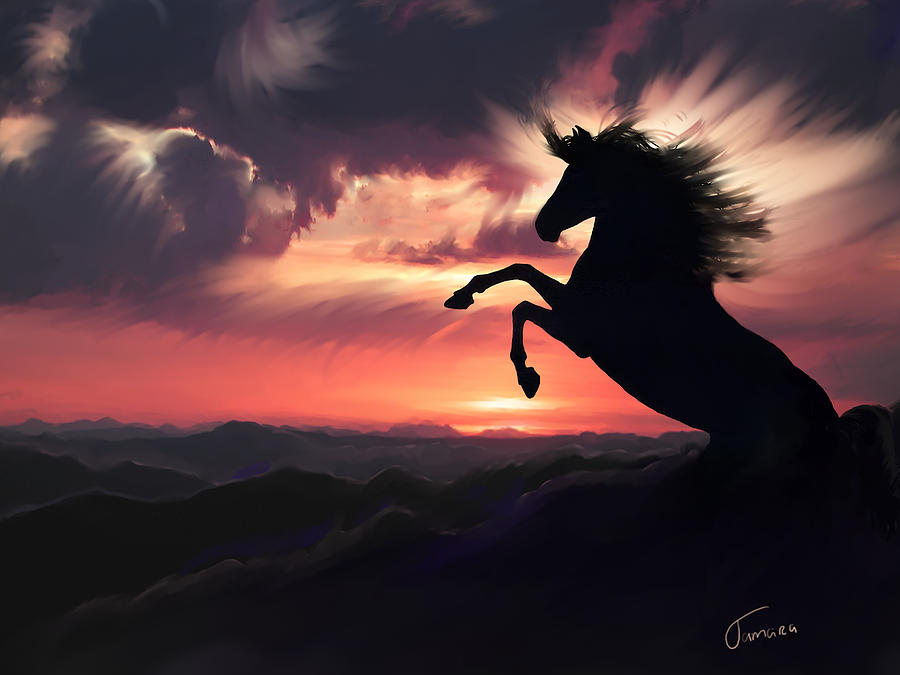The image features a dramatic silhouette of a rearing horse, depicted in black as it leaps off its hind legs with its mane streaming back. The horse, positioned on the right side of the composition, is shown in a dynamic pose with both front legs raised – the left leg slightly bent beneath the right. In the background, the vibrant orange hues of a setting or rising sun illuminate the scene, creating a stark contrast with the dark silhouette. Above, streaks of gray clouds scatter across the sky, while below, a series of mountain ranges, rendered in black and shades of gray and purple, add depth to the landscape. The artist’s signature is visible in the lower right corner, confirming this as a painting rather than a photographic or computer-rendered image. The overall effect is one of wild, untamed beauty, captured at a moment of powerful motion against the tranquil yet vivid backdrop of a twilight or dawn sky.